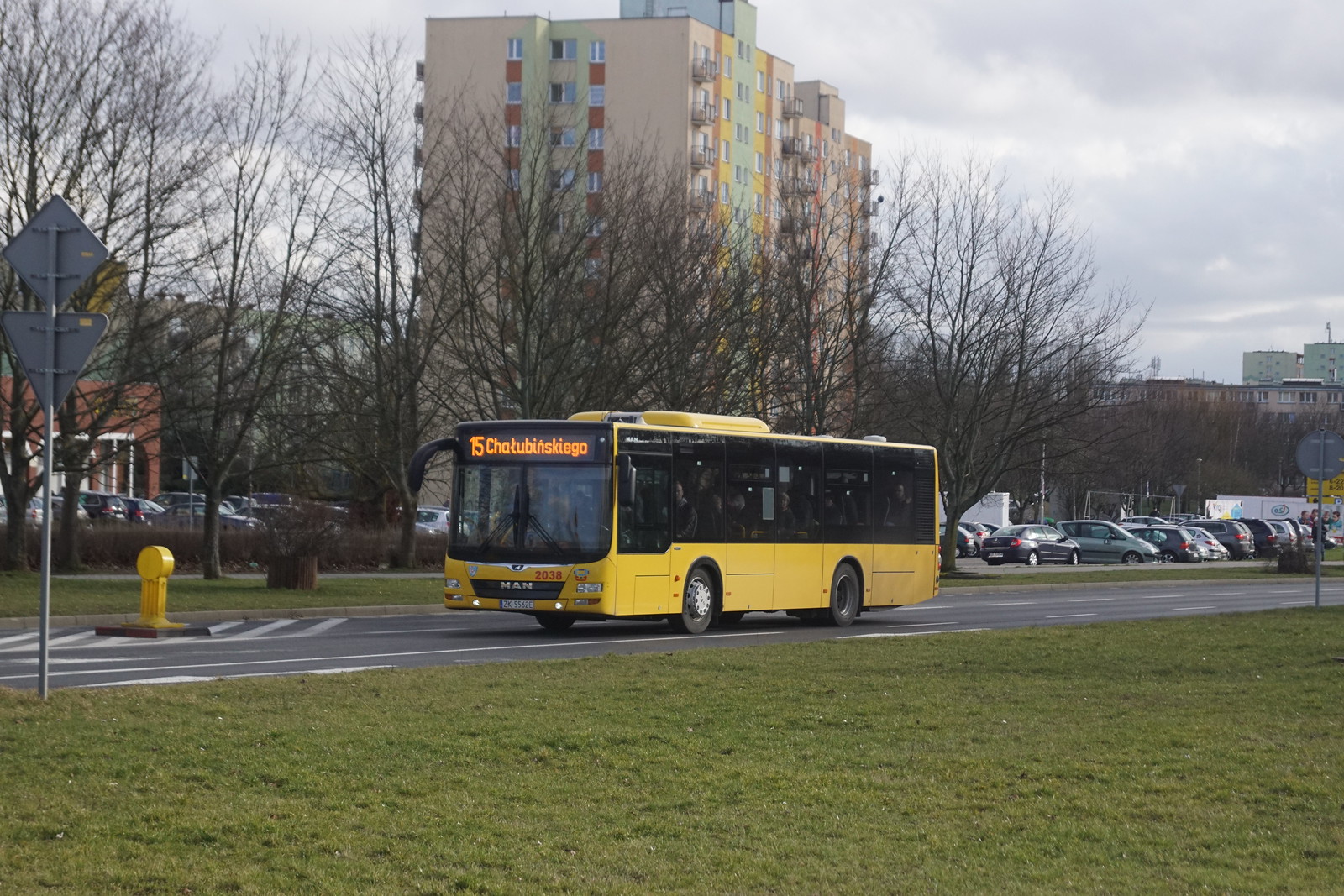The image captures a scene on a cloudy, overcast day in what appears to be an Eastern European city, as suggested by the bus's destination display reading "15 Chatubumskiemgo." The primary focus is a yellow public transportation bus with large shaded windows, a digital display at the front, and the number 15 prominently visible. The bus is traveling down a gray asphalt road with white lane markings and flanked by short grassy areas. In the background, a high-rise apartment building with multicolored trim—featuring yellow, blue, and red stripes—stands out prominently. Several other buildings of varying heights, in brown, green, tan, and brick hues, are visible, along with a notable amount of parked cars. Several leafless trees stretch across the scene, adding to the urban wintery atmosphere. The area appears to be a mix of residential and commercial properties, with multiple street signs punctuating the scene.